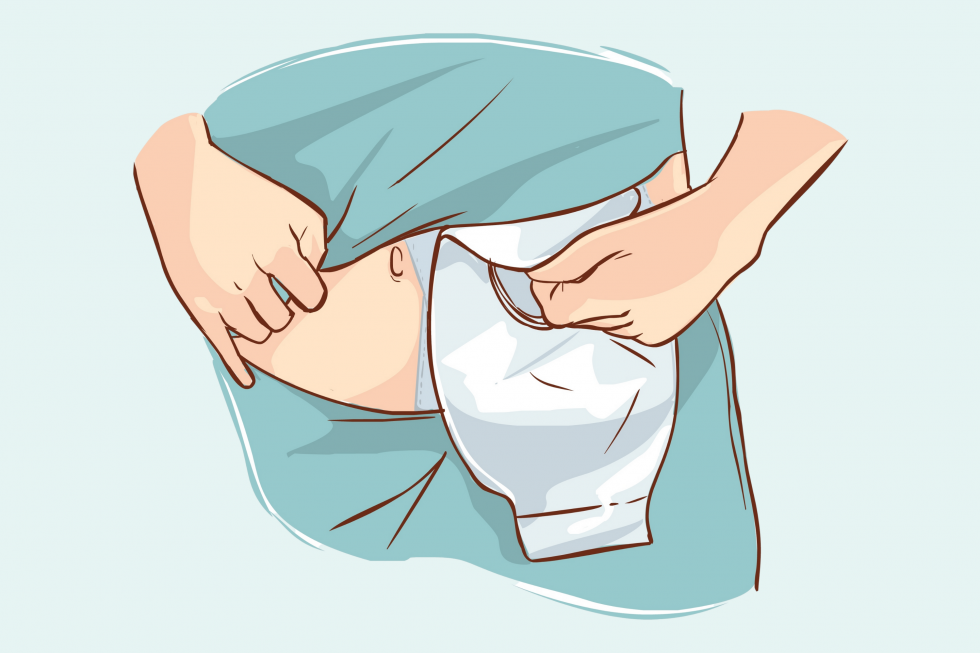The image is a detailed graphical or clip-art illustration depicting the midsection of a person, likely a woman or patient, in a hospital setting. The person is wearing a blue hospital gown, with one hand lifting the gown to expose the belly area. The other hand is handling a white, transparent bag that appears to be placed on the stomach, possibly indicative of a medical procedure such as an ostomy. Additionally, there is a bandage visible on the left side of the belly. The background is a light blue or sea-green color, providing a clinical and sterile setting to the image. The perspective shows the person from the belly button down to the hips, emphasizing the medical context and the handling of the medical equipment.